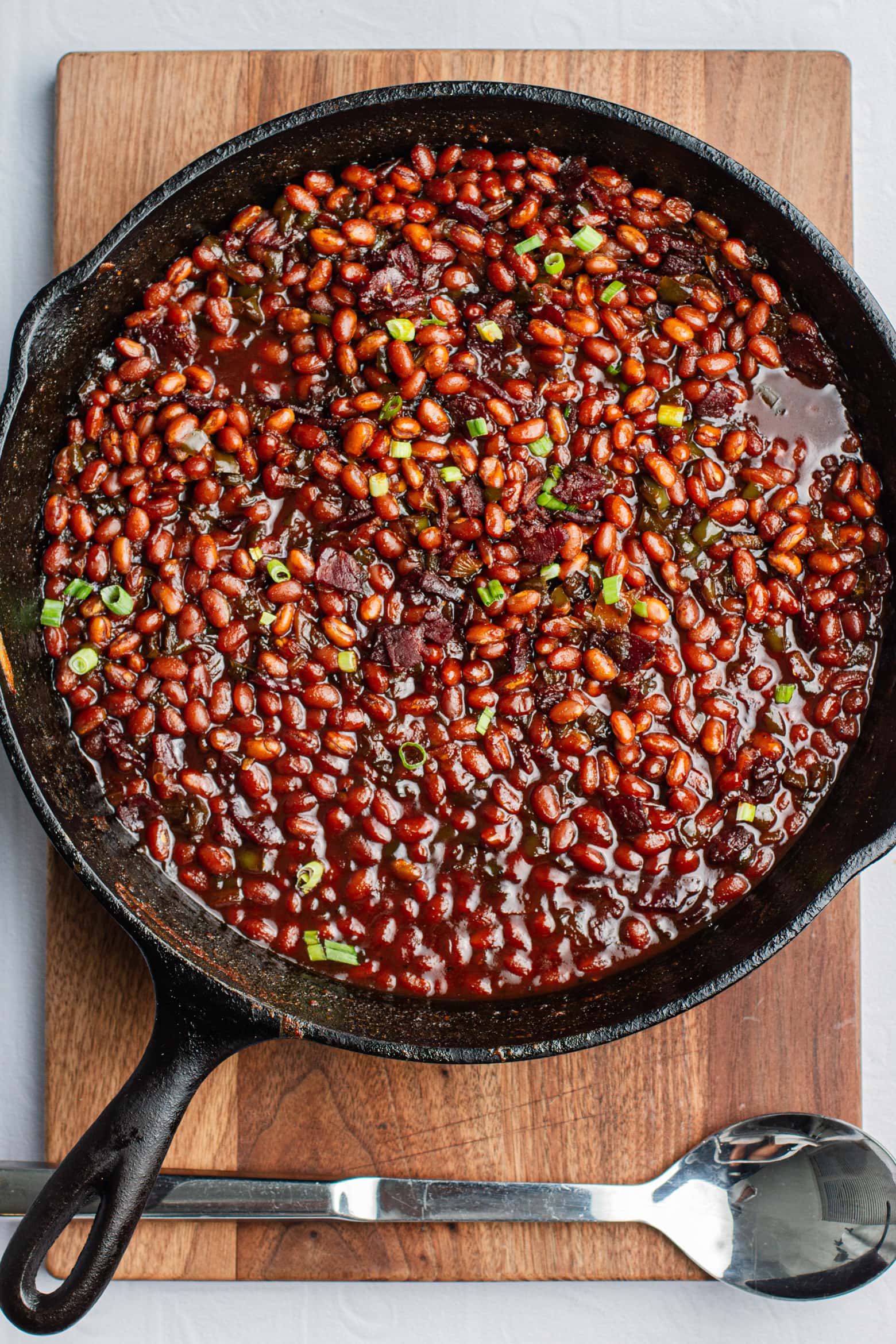The overhead color photograph depicts a close-up of a cooking scene centered around a large black cast iron skillet. The skillet is filled with a vibrant assortment of beans, possibly pinto or red beans, bathing in a rich sauce. Scattered among the beans are small slices of green vegetables, likely chives, but possibly bits of asparagus or celery, providing a burst of fresh color. This hearty dish could be a type of chili or bean stew.

The skillet is placed securely on a sturdy wooden cutting board, which rests atop a gray surface. At the bottom of the photograph, a large, reflective metal spoon is positioned, likely used for stirring or serving the dish. The image is well-lit, showcasing the textures and colors of the ingredients clearly, invoking a sense of warmth and home-cooked comfort.